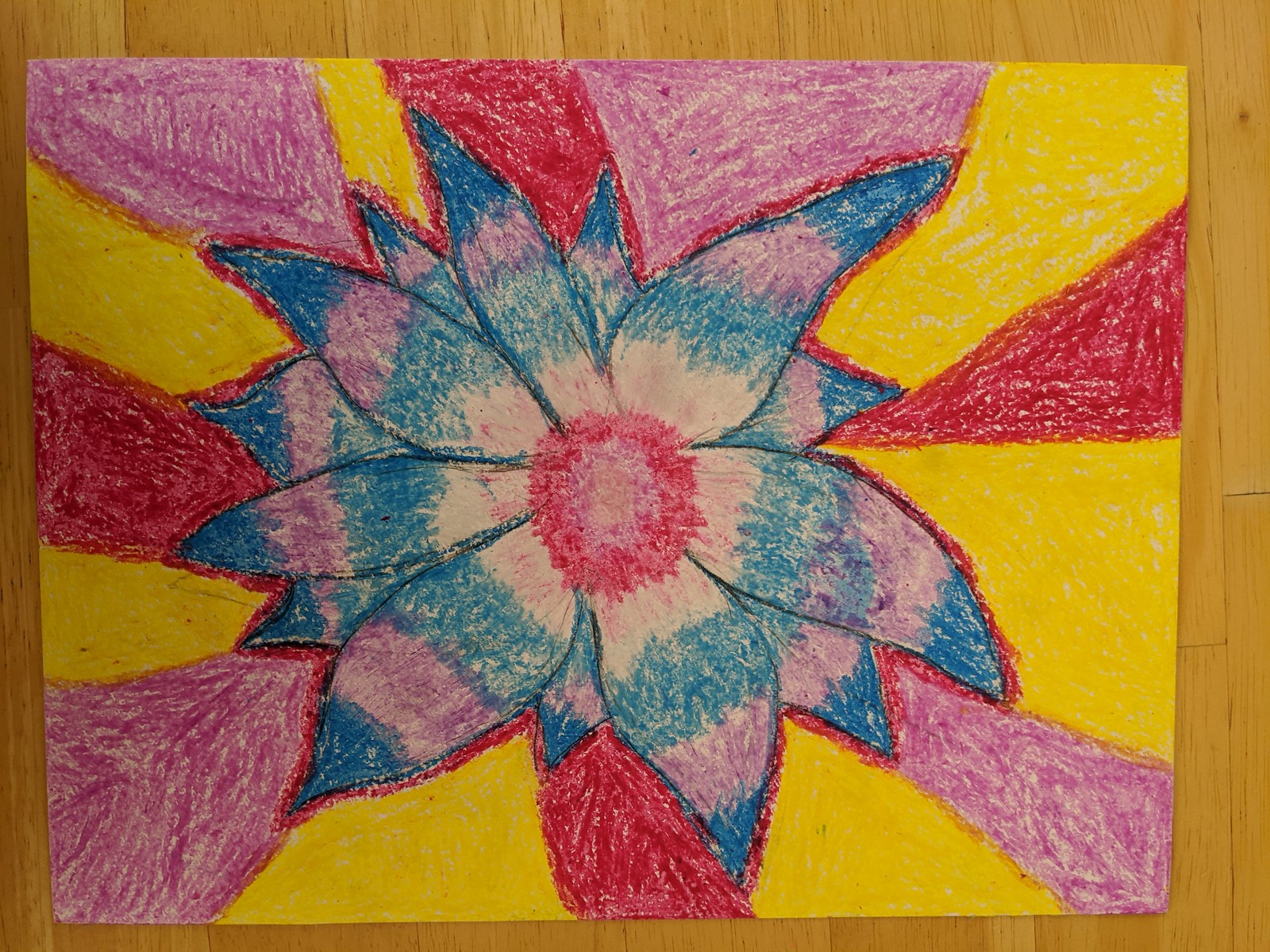The image showcases a vibrant crayon drawing placed on a hardwood floor. At the center of the drawing is a flower with a rich red core, interspersed with pink details signifying seeds or pollen. Surrounding this center, the petals radiate outwards, transitioning from pink near the core to blue, further blending into purple and then dark blue at the edges. The flower is adorned with approximately 15 to 20 leaves, each bursting with energy-like colors. These emanating colors follow a sequential pattern of yellow, red, yellow, pink, and then repeat, creating an impression of dynamic energy surging from the petals. The interplay of hues and the detailed transitions between them highlight the intricate, energetic, and lively essence of the drawing.